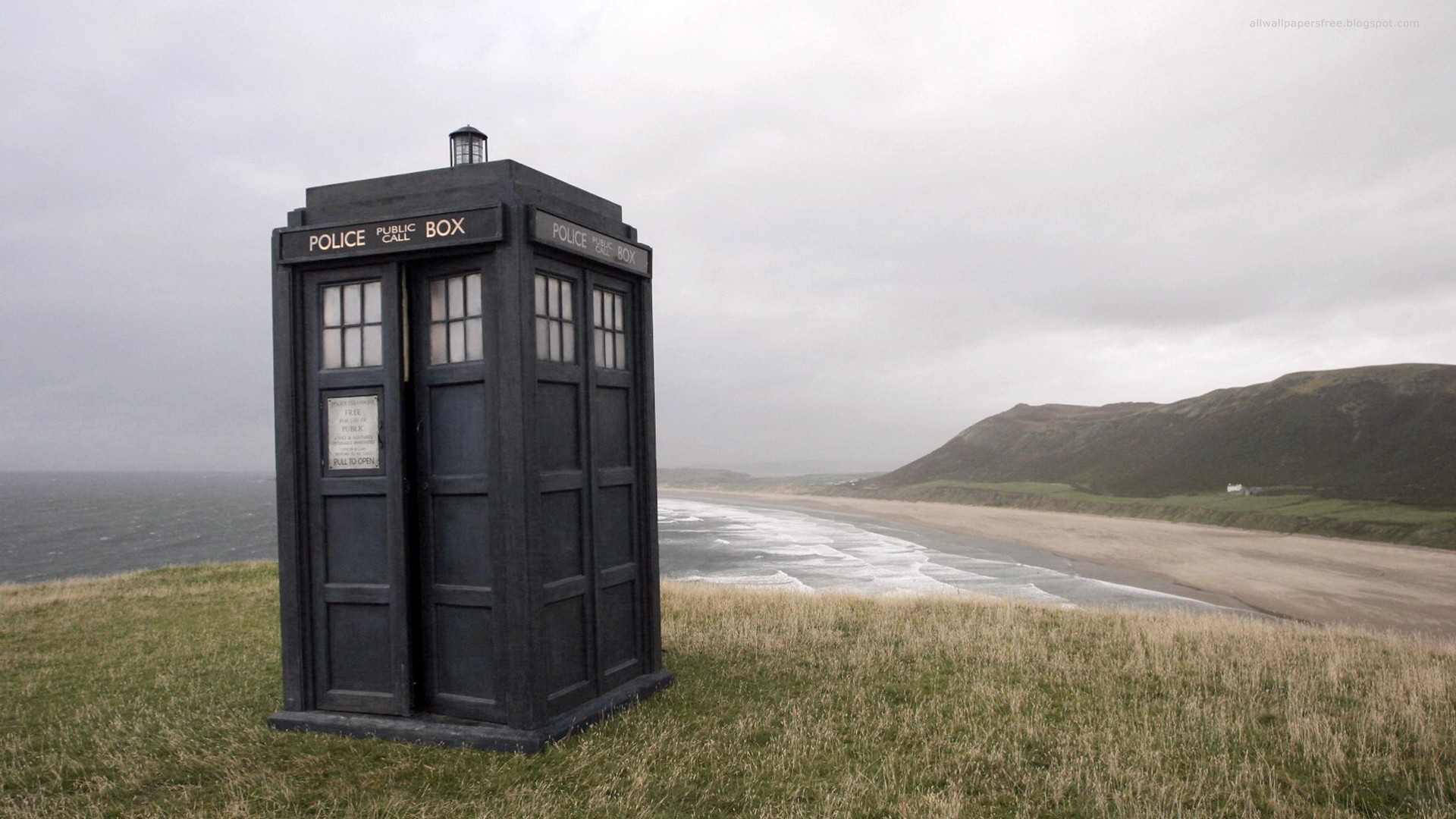The image depicts a misty and foggy beach scene characterized by a muted color palette. In the foreground, there's a mix of yellowish, dead grass and patches of light green grass on a small hill. Dominating this area is an old-fashioned black police public call box, resembling a phone booth, with white windows and a small light on top. The words "Police Public Call Box" are prominently displayed at the top, though partially obscured. The beach stretches out behind the hill, featuring beige sand leading to a gray, misty ocean, with gentle waves lapping at the shore. In the distance, mist-shrouded mountains and tall hills, primarily dark brown with occasional muted green patches, rise away from the shoreline. The sky overhead is predominantly gray and cloudy, contributing to the overall cold and hazy atmosphere of the scene.